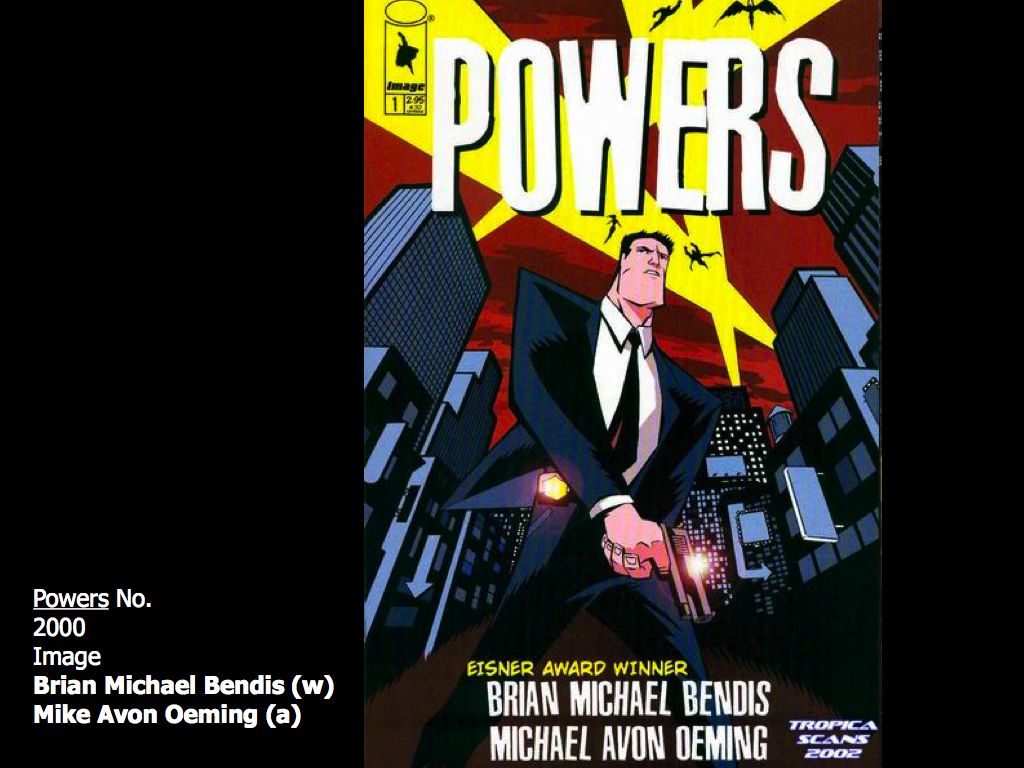The image showcases a vividly illustrated comic book cover set against an all-black background. Dominating the center of the composition is the cover art of the comic book "Powers." In large white text at the top, it proudly displays the title "POWERS." Centered within the image is a striking illustration of a white male character with a thick jawline, dressed in a suit, white shirt, and black tie, and holding a pistol. The perspective gives an upward view of the man as he walks down a city street, bordered by towering high-rises illuminated by yellow searchlights. Scattered within these searchlights are at least four small illustrations of people flying. Adding to the detailed cityscape, several bugs or bats can be seen flying underneath the beams. 

On the top left corner, the image logo is present with the number one, indicating it is issue number one. Further text includes “Eisner Award winner Brian Michael Bendis” at the top, while the bottom left corner features the text “Powers Number 2000 Image,” followed by the creators’ names, “Brian Michael Bendis W. Mike Avon Oeming A.” The palette includes nuanced shades like black, white, yellow, maroon, brown, and light blue, enhancing the comic book's dramatic and noir-like aesthetic.